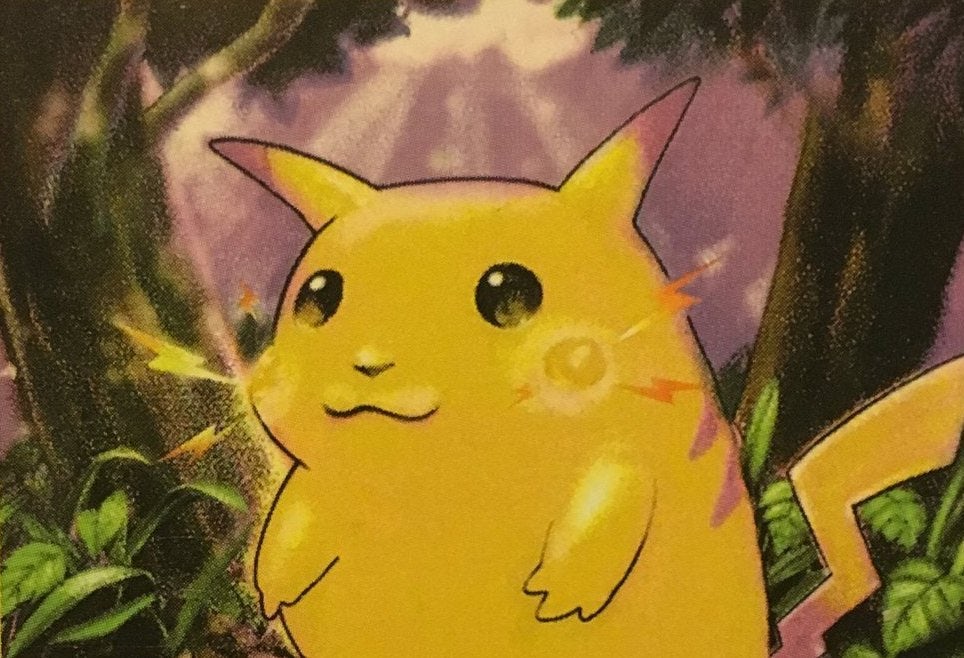This image is a beautifully detailed, hand-drawn cartoon illustration inspired by the Pokémon franchise, featuring Pikachu as the focal point. The scene is set in a mystical forest with a striking, purple-hued sky that gradually shifts to reveal some white clouds, through which the sun is breaking, casting its rays warmly on Pikachu's face. 

Pikachu, prominently positioned in the foreground, captures immediate attention with his vibrant yellow fur and signature lightning bolt-shaped tail, accented with purplish pink markings. His body is adorned with orange lightning zigzags, adding dynamic energy to his appearance. Pikachu’s expressive, large black eyes and pointed ears—tipped with a unique pinkish-purple tint—contribute to his endearing charm.

The background features two brown trees flanking Pikachu, each leaning slightly outward towards the edges of the image, balancing the composition. Scattered on the ground is a layer of colorful foliage, enhancing the forest setting. With its imaginative depiction and intricate details, this artwork offers a fresh and enchanting take on the beloved character, Pikachu.